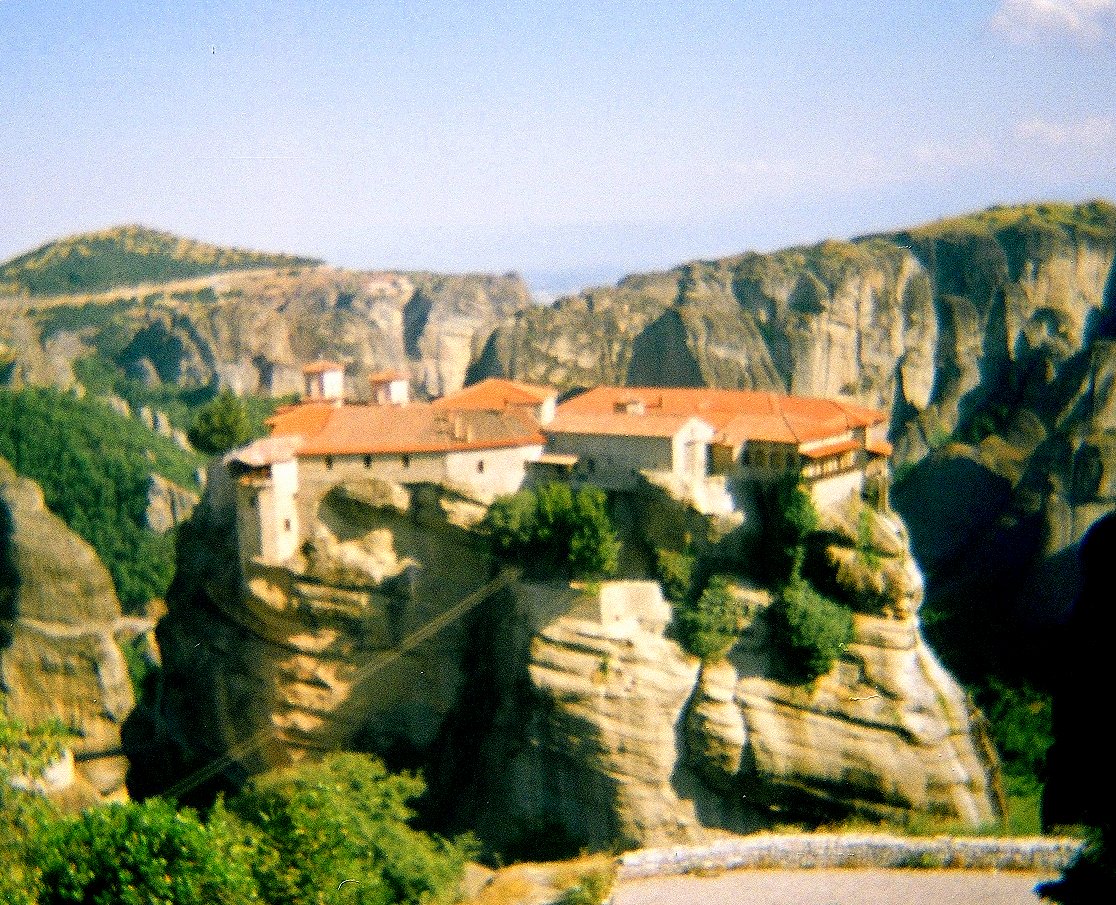This image captures a slightly grainy, outdoor scene of a dramatic landscape dominated by rocky cliffs and lush greenery. Dominating the center of the scene are a series of buildings, resembling large houses or perhaps a castle, characterized by their orangey-red roofs and beige or white walls. These structures sit atop a prominent rock precipice, surrounded by steep drop-offs and a verdant valley below. The rock formation is beige, punctuated by vibrant green trees that partly cover its rugged surface. To the sides, more cliffs can be seen, creating a scenic backdrop. The sky above is a clear blue, decorated with some puffy white clouds in the upper right corner, adding to the picturesque quality of the scene. A tower is visible on one side of the main structure, further enhancing the architectural interest of the buildings.